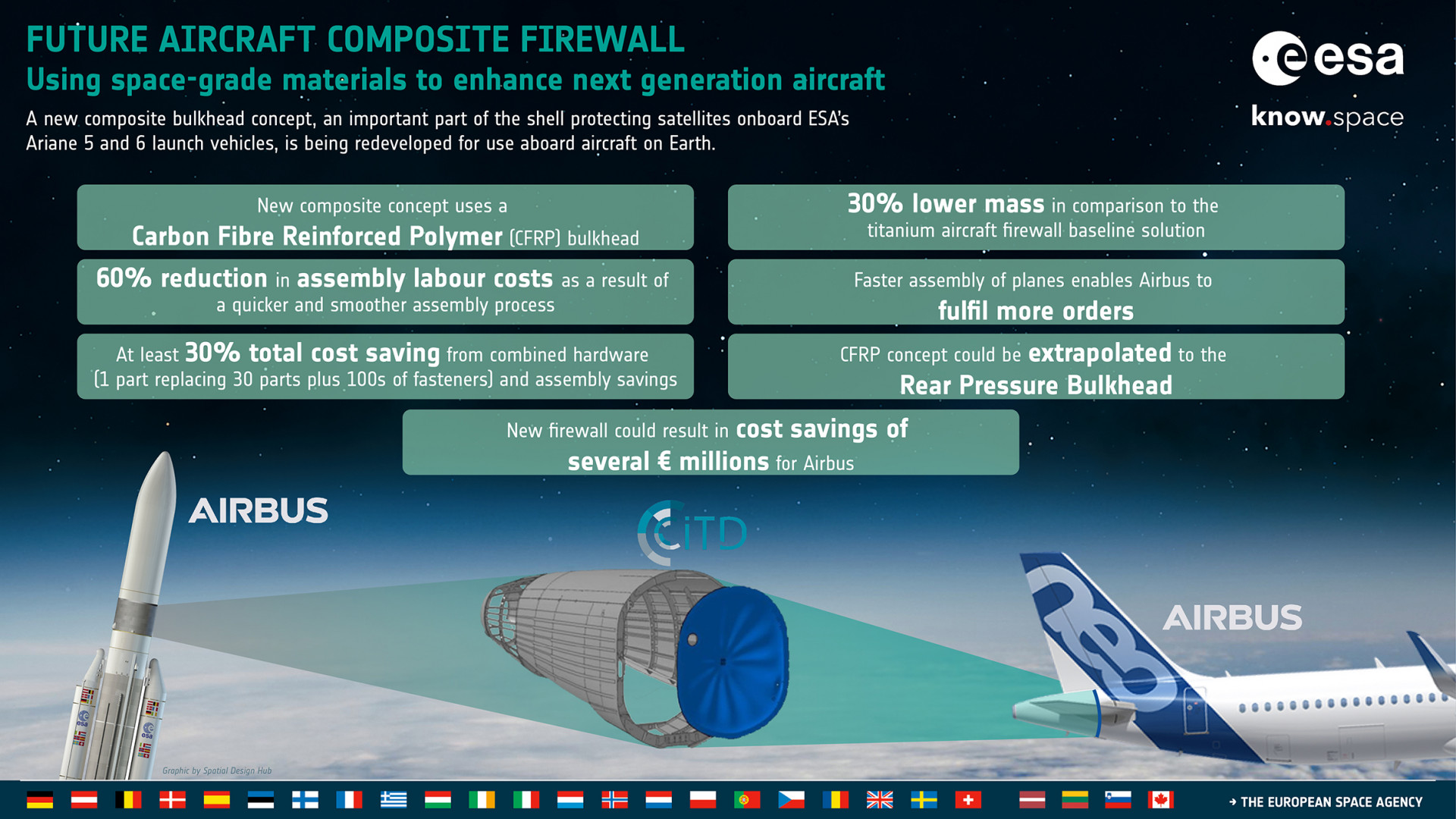The image showcases a concept advertisement for aerospace innovations, combining elements from space and aviation sectors. At the top left in green lettering, it prominently displays the title "Future Aircraft Composite Firewall Using Space-Grade Materials to Enhance Next-Generation Aircraft.” Directly below, in white lettering, it reads, "A new composite bulkhead concept, an important part of the shell protecting satellites onboard ESA's Ariane 5 and 6 launch vehicles, is being redeveloped for use aboard aircraft on Earth." The design effectively integrates multiple visual elements and informative blocks. There are green rectangular sections with white text detailing key statistics, such as “carbon fiber reinforced polymer” and a “60% reduction in assembly labor costs.” 

Further down, the image features illustrations: on the left, there is a picture of a rocket with the label "Airbus," while on the right, there is a partial image of an Airbus airplane displaying the tail and wings. Additionally, a digital illustration of the composite firewall is situated between these images. The right side of the image contains the logo "ESA" with a distinctive red dot, along with international flags lining the bottom edge. At the very bottom, the European Space Agency's full name is mentioned. This comprehensive visual presentation emphasizes the collaboration and technological advancements aimed at revolutionizing the aerospace industry.